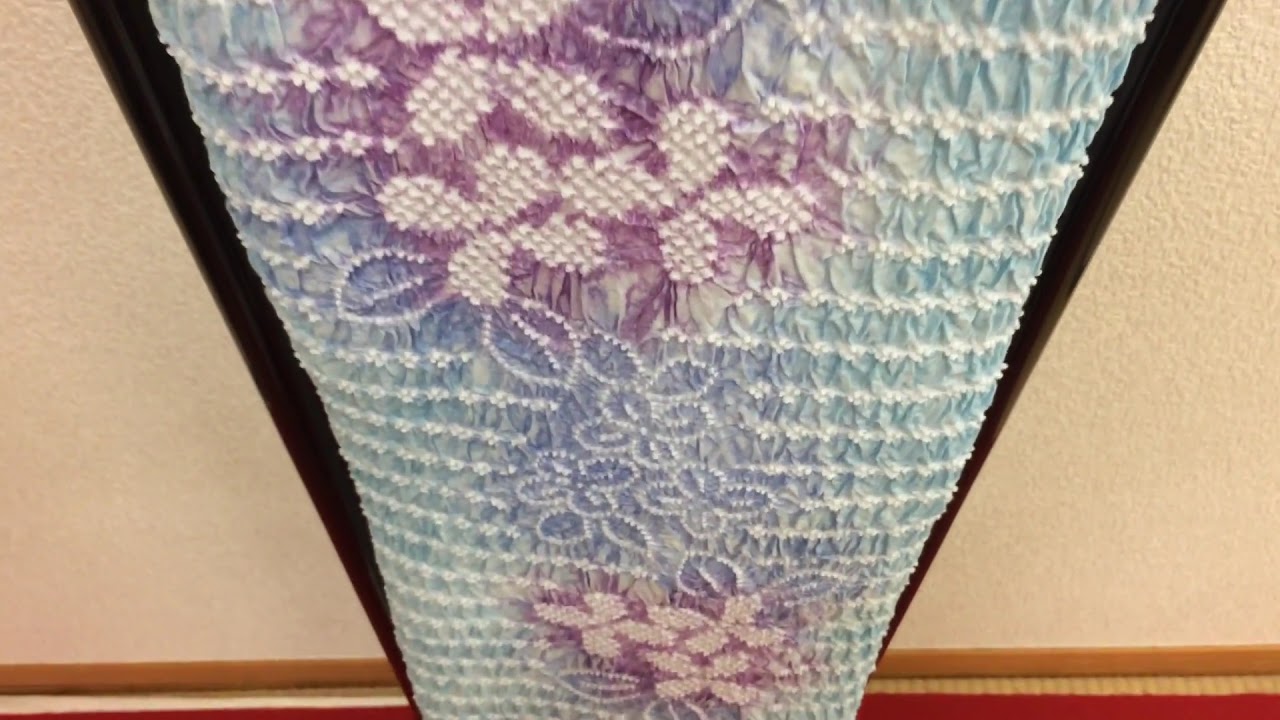The image displays an ornate, vertical strip of fabric or tapestry hanging on a wall, centered in the frame. The fabric, which stretches nearly the entire height of the image, features a heavily textured and pleated pattern with intricate designs that include what appear to be small pearls, embroidery, and stitching. A prominent element is a series of purple and white flowers arranged in a tie-dyed effect, alongside outlined leaves and four-leafed plants. Three additional white, petal-shaped flowers on a purple background can be seen towards the bottom of the fabric. The fabric runs from a wider top to a narrower bottom. The background consists of a black border, and the piece is hung against a tan wall, with a red carpet visible at the bottom of the image, reinforcing the impression that the tapestry is mounted vertically.